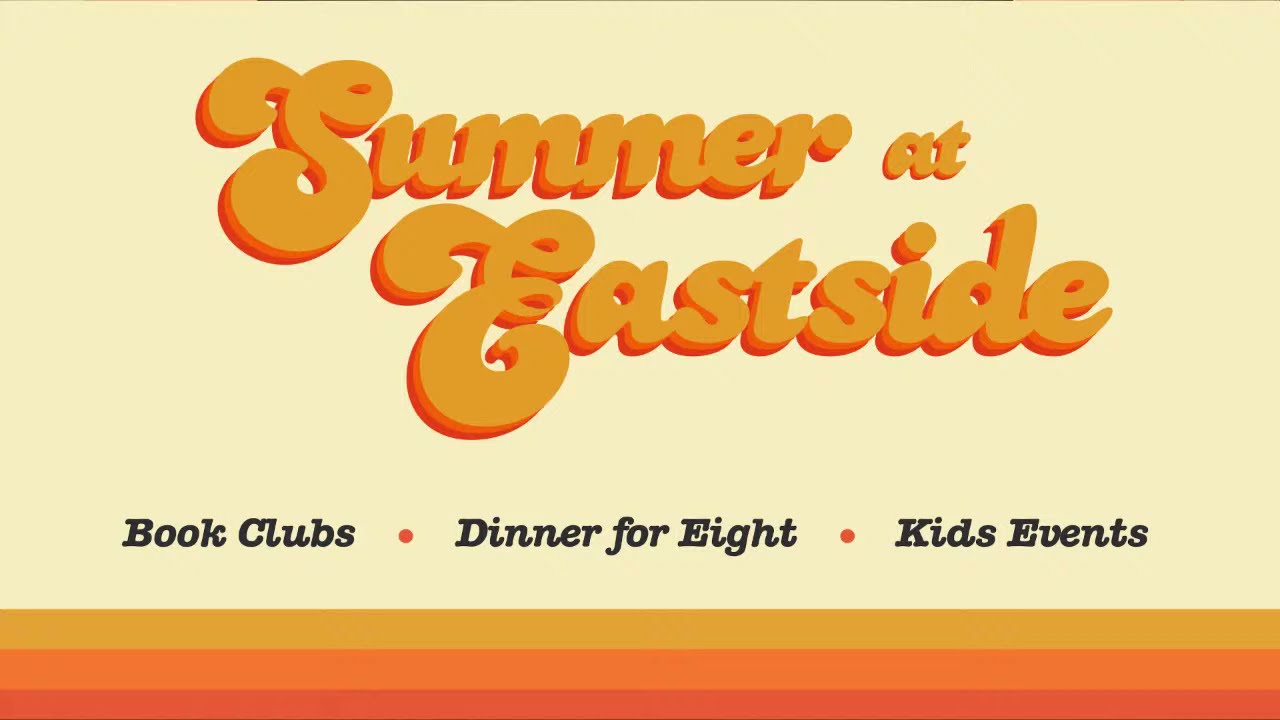The image is a stylized flyer resembling a 70s theme, featuring a creamy white background with an eye-catching text and colorful accents. Prominently displayed in a groovy, cursive font with orange and red drop shadows, the text reads "Summer at Eastside" with "Summer" being larger than "at" and "Eastside" matching "Summer" in size. The text gives a 3D effect in an orangey-mustard hue, occupying two lines in the upper-middle section of the flyer. Below this, in capitalized black block letters, are the phrases "Book Clubs," "Dinner for Eight," and "Kids Events," each separated by an orange-red dot. The bottom portion of the flyer is adorned with three horizontal stripes: the top stripe is mustard yellow, followed by orange, and the bottom-most stripe is red, adding a vibrant border to the flyer. The overall aesthetic combines a warm, retro vibe with modern event information.